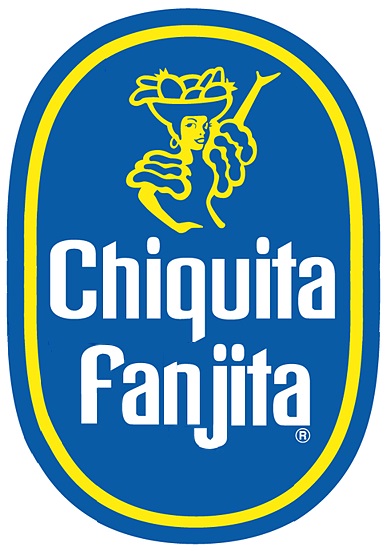This image features a large blue sticker, commonly seen on bananas, with a yellow oval border. At the center of the sticker is the iconic Chiquita brand logo, depicting a confident woman in yellow, with gold hoop earrings and an expression with her mouth open and eyes looking to the left. She balances a basket of fruit on her head, which includes a pineapple and several bananas. One of her hands is on her hip, while the other is stretched out with an open palm. The sticker's text reads "Chiquita Funjita," with a registered trademark symbol, a white "R" inside a white circle, situated beneath the final letter "A." The overall design is reminiscent of an egg shape and vividly captures the essence of the brand.